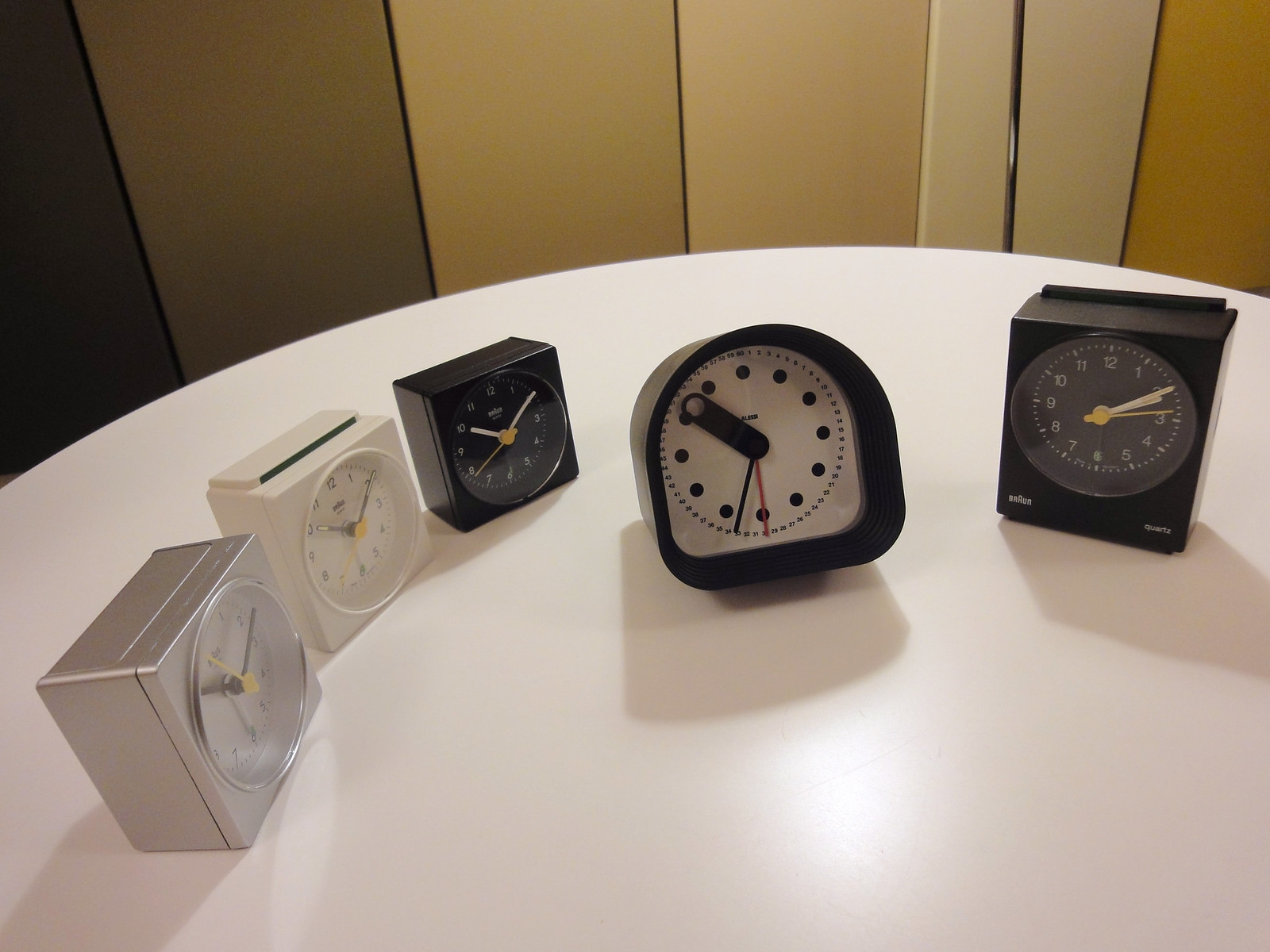This photograph captures a striking arrangement of five clocks neatly displayed on a glossy, round white table that appears to have a laminate finish. Behind the table, the backdrop features paneling in various shades of beige and gold, adding a touch of warmth and elegance to the scene. Notably, a wire descends the wall and disappears under the table, introducing an element of industrial modernity.

Starting from the left, the first clock is a sleek, silver, perfectly square timepiece. It houses a round analog face with conventional numbers, black hour and minute hands, and a vibrant yellow second hand. The second clock mirrors the design of the first but sports a white plastic casing instead of silver. Similarly, the third clock is identical in functionality and design but is encased in black plastic. Due to the black background of the clock face, the numbers and the hour and minute hands are white, providing a stark contrast that enhances readability.

The fourth clock diverges from the theme, presenting an elegant arch shape with a rounded top and a flat bottom. Its black casing encircles a white face inset about half an inch, creating a subtle shadow effect that emphasizes its modern design. Despite its contemporary appearance, it remains analog, featuring a bold, elliptical hour hand with a hollow end, a thin black minute hand, and a delicate red second hand. Instead of numbers, dots represent the hours, while tiny minute numbers outline the perimeter.

The final clock returns to the square shape but is slightly more rectangular in height. It also has a black face with white numbers and hands, maintaining the monochrome theme. The minute and hour hands are white, while the second hand adds a pop of yellow. This clock includes a brand name positioned on the bottom left and additional, unreadable writing on the bottom right, adding a hint of exclusivity and precision to its design.

Together, these clocks form an intriguing visual tableau, blending uniformity in design with subtle variations in color, shape, and detailing, set against a sophisticated, neutral background.